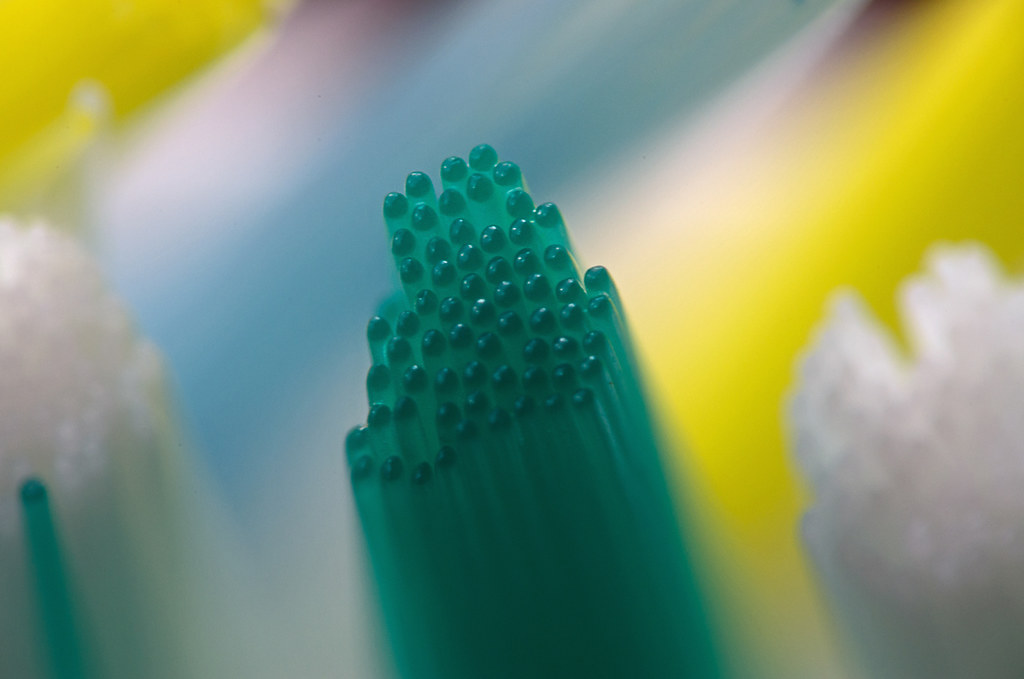The image features a close-up of a mysterious object that is difficult to identify, predominantly composed of medium to dark green, bristle-like or tubular strips bundled tightly together, each topped with a darker green, blunt, rounded cap. The focal point is sharp at the very top of this central cluster, while the sides and the background are blurred. Flanking this central green bundle are two similar-looking groups of white objects that mirror the green formation, although heavily blurred. The background fades into a blurry gradient of wide, slanted streaks of color, transitioning from yellow in the upper left corner, to light blue on the right, then back to yellow again at the far right, interspersed with hints of purple accents near the top of the image. While it remains ambiguous whether the image represents a natural or technological subject, the detailed arrangement and coloring evoke an intricate and aesthetically structured composition.